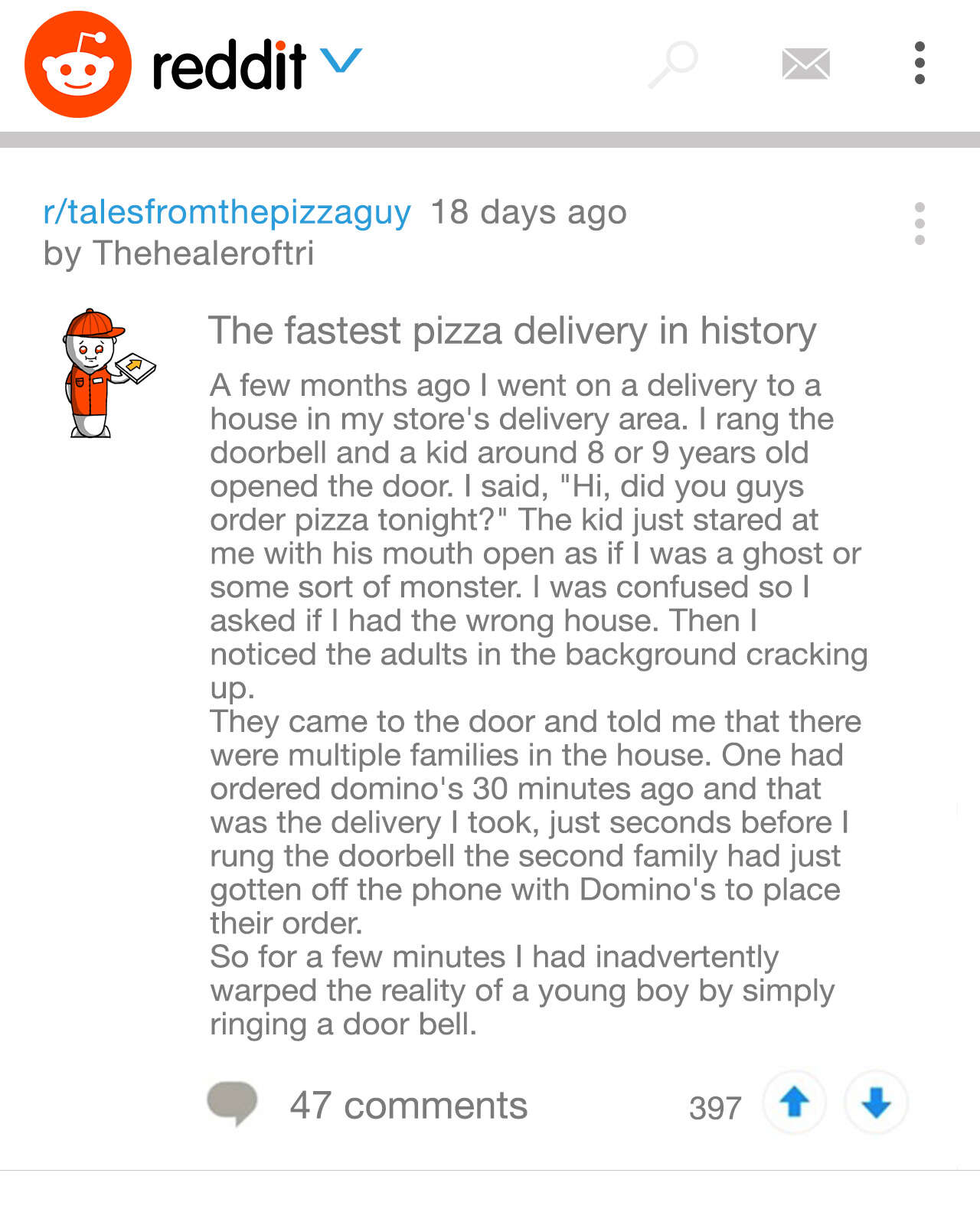**Caption:**
An image from a Reddit page featuring the r/talesfromthepizzaguy subreddit, posted 18 days ago by the user "TheHealerOfTRI." The post, titled "The Fastest Pizza Delivery in History," narrates a humorous incident that occurred during a pizza delivery. The story describes how the delivery driver rang the doorbell of a house, only to be greeted by a wide-eyed, speechless child, presumably aged eight or nine. The driver, realizing something was off, asked if they had the right house. This prompted laughter from the background adults, who explained that there were two families in the house. One family had ordered Domino's pizza 30 minutes prior, and their delivery had just arrived. Meanwhile, the second family had just placed their order with Domino's, creating a moment of confusion for the young boy when the doorbell rang. The post garnered considerable engagement with 47 comments and 397 upvotes, capturing the humorous essence of an unexpected and amusing delivery coincidence.